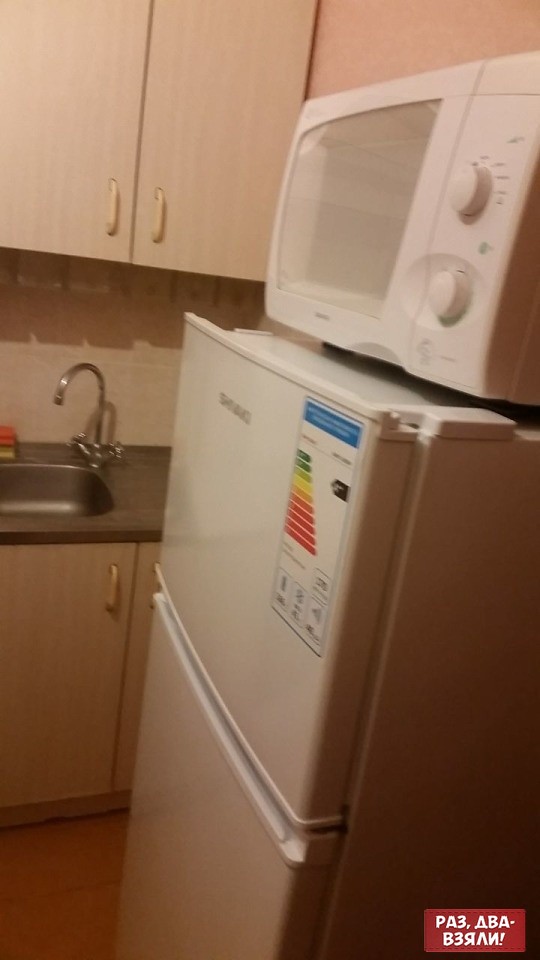This vertically cropped, low-resolution color snapshot features a cluttered kitchen corner dominated by a diagonally positioned, smaller-sized, white refrigerator stretching from the bottom left to the upper middle of the image. The refrigerator sports a label with a schematic, cascading colored graph ranging from green to maroon red, though the text is unclear. Atop the refrigerator sits an older-style white microwave with a glass door, two large round white dials for time and heat settings, and a small green button in between. In the background, a kitchen counter with a stainless steel sink and a silver faucet is visible, adorned with a few sponges. The cabinetry above and below the counter is wood with light-colored handles. A small red rectangle with cryptic white text, including characters like "PA3" and "BA-B3," occupies the lower right corner of the image.